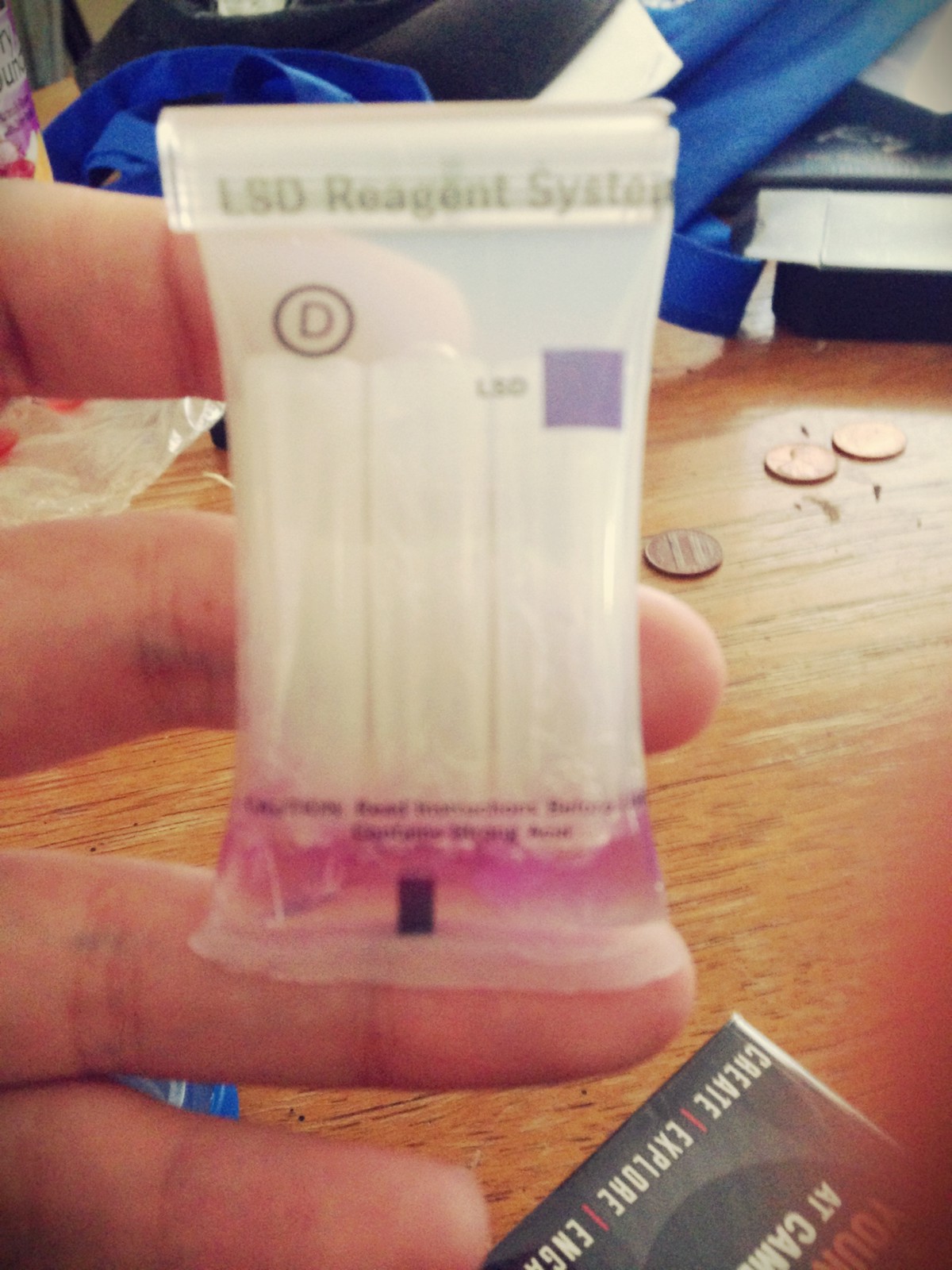The image depicts a close-up of a person's left hand holding a small, opaque white plastic package used for drug testing, specifically an LSD reagent system. The package has a distinct "LSD reagent system" label at the top along with a black "D" encircled. A little purple square with "LSD" written inside is also visible on the left side of the package. Inside the clear package, various small opaque test tubes can be seen, some of which have been broken to produce a pinkish-purple liquid at the bottom. The person's hand, prominently featuring dark veins, is positioned over a brown wooden table. On the table, there are three scattered pennies—one showing tails and another heads—a partially visible book with words like 'create' and 'explore' on its black and red cover, alongside other assorted items such as a blue bag and additional books and plastic packaging in the background. The image captures a detailed snapshot of the testing package and its surroundings, providing a thorough context for the items in the scene.